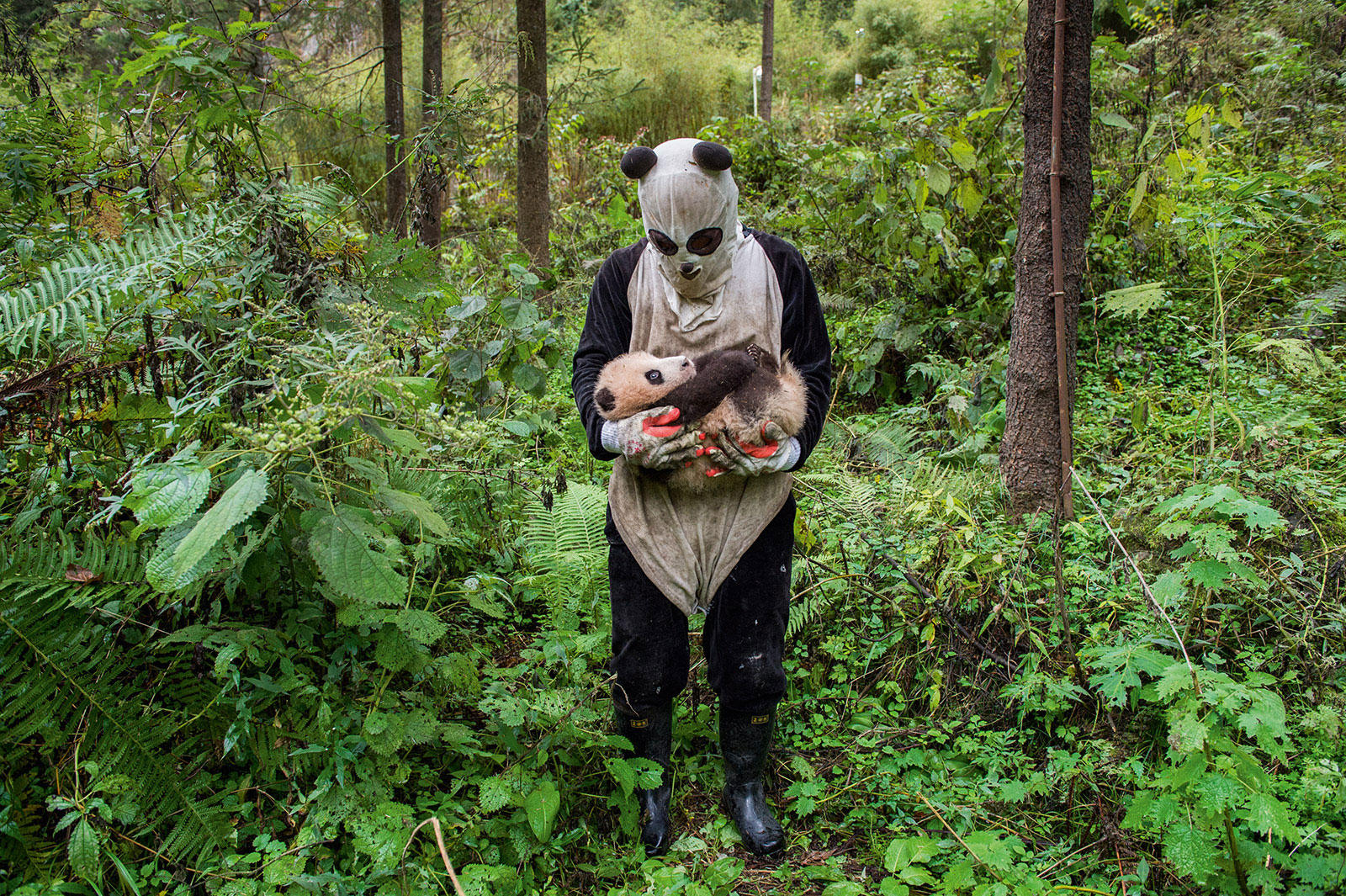In this odd yet captivating image, a man dressed in a full-body panda costume stands deep within a vibrant, green jungle. The man is fully covered in a panda suit that features big black eyes, distinct black ears, black arms, legs, and a fluffy white torso, complete with a hood that covers his head like a panda mask. His hands are gloved to resemble panda paws, and he wears rubber boots suited for the dense forest terrain. Cradled gently in his arms is a small, curled-up baby panda bear, which has white fur with black arms and appears slightly dirty, giving it a light brown hue. Surrounding them is a lush, green forest brimming with various types of vegetation, including tall trees, ferns, and shrubs, creating an untouched, pathless wilderness. This attire and setting hint that the man may be a zookeeper, likely in an Asian conservation area, where dressing as a panda helps young pandas feel safe and nurtured, mimicking the presence of their mother.